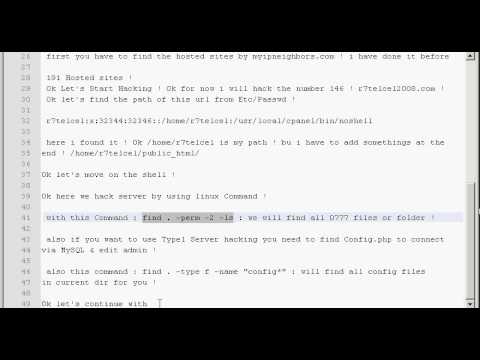The image displays a piece of lined paper with black borders at the top and bottom. The paper has poor resolution, making the text appear as if it was typed on white paper. Each line of text is numbered, and the visible portion includes lines 21 through 49. 

The content on the paper begins with instructions: "First, you have to find the hosted sites by myipneighbors.com. I have done it before." It then skips a line and continues with: "151 hosted sites." The next line appears to start with an attempt at typing “hacking,” but only parts of the word are discernibly spelled out as "h-a-o-k-i-n-g." It goes on to say, "Okay, for now, I will—" followed by a jumbled mix of numbers and a URL, "r7teloe1n008.com".

Further down, the text attempts to outline a method to find the path of a URL, mentioning directories like "/etc/". This section is fragmented and interrupted by another skipped line, followed by a seemingly random string of alphanumeric characters. It concludes with a partially clear element: "Here I found it," followed by instructions to navigate directories, including mentions of "i7telce," "/home/," and ending with "/public_html/."

Overall, the document appears disorganized and is potentially related to website hosting files and paths, though the exact context remains unclear due to the fragmented nature of the text.